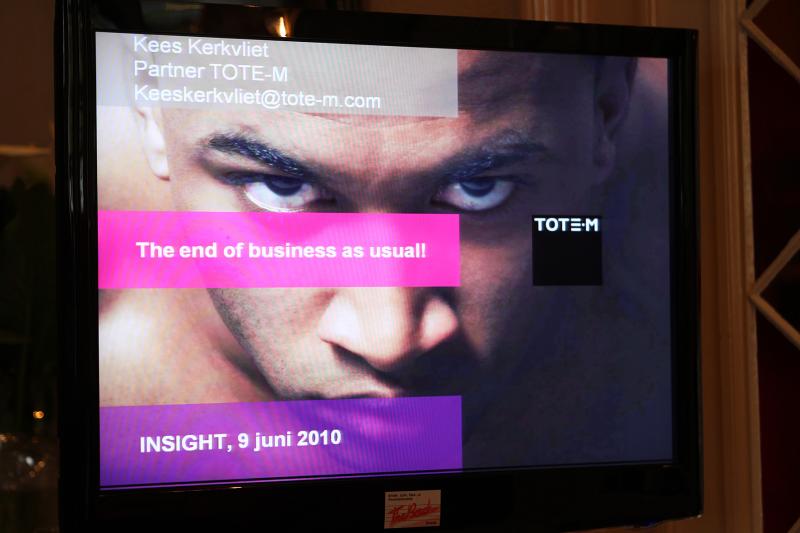This detailed description combines and refines elements from the provided captions:

The image depicts a photo of a screen, likely a flat screen TV or monitor, mounted against a wall. The background is a mix of brown and white shades, with a hint of a window on the right side and dark sections on the lower left, possibly showing reflections or objects like a glass cup. The screen itself is bordered in black and displays a striking close-up of a black man's face. His head is tilted downwards while his intense eyes look directly up into the camera, giving him a serious or even ominous expression.

There is noticeable glare from a flash in the upper, slightly left-of-center part of the screen. Overlaid on the screen are several colored banners with white text. In the top left, within a light gray banner, the text reads "Keese Kerkivliet, Partner, Totem" followed by an email address. Below this, a pink banner exclaims "The End of Business As Usual!" To the right side of the screen, a black square features the Totem logo. At the bottom left, a purple banner reads "Insight 9 June 2010." Additionally, there appears to be a small white sticker with red text on the bottom of the TV itself.